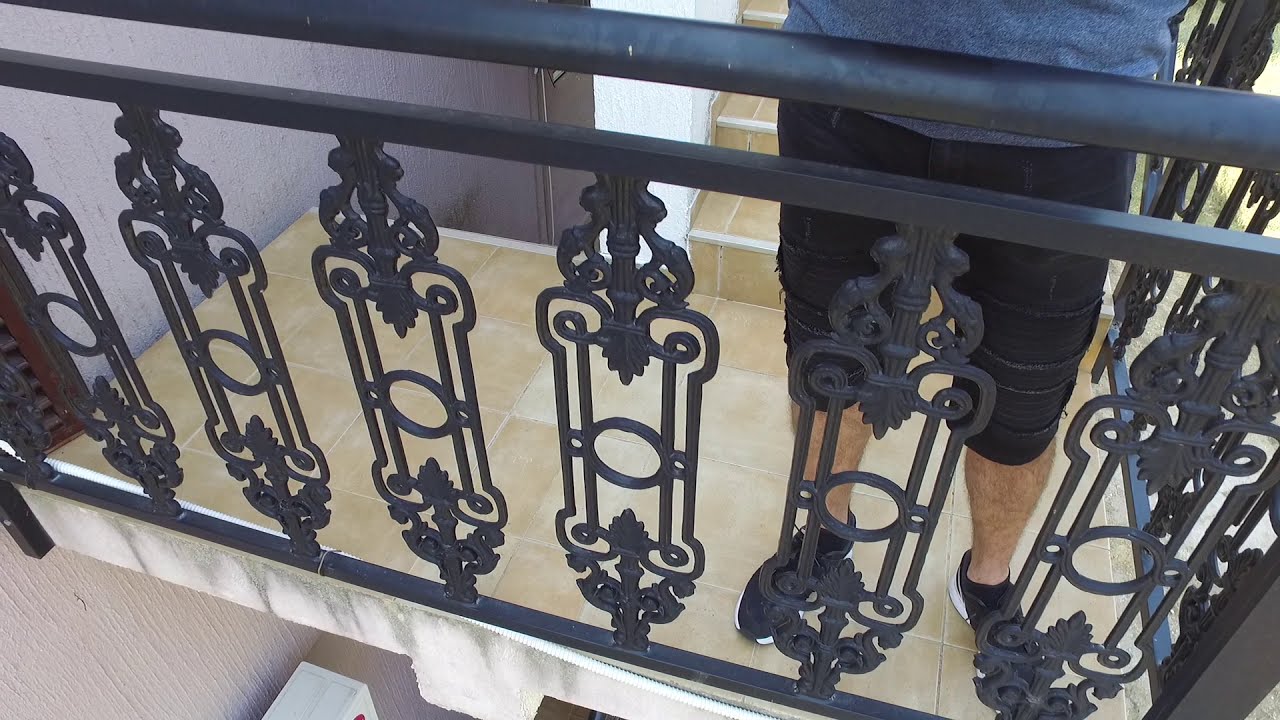In this photograph, we see the lower half of a Caucasian man leaning against a black wrought iron staircase banister with an antique, Art Deco style. The image is viewed from above, showing him standing on the second floor of a three-story building. The man is dressed in a light blue t-shirt, black shorts reaching his knees, and dark sneakers. He is positioned on tan-colored tiles, facing the camera. Behind him to his right is another flight of stairs descending to the floor below. The walls are painted gray, and the dark railing of the adjacent staircase is visible, framing the limited view from the man's stomach down to his feet.